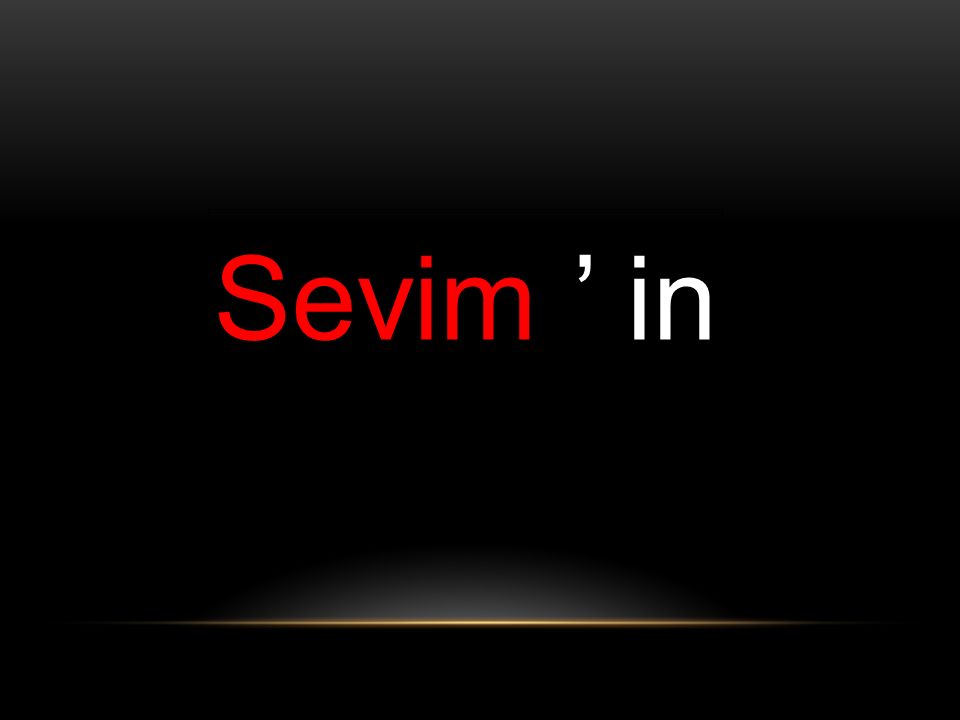The image features a primarily black background, accentuated by a gradient effect along the top transitioning from a lighter black to pure black. Centered on the black background is the text "SEVM, IN," with "SEVM" in bold red font and "N" in white, accompanied by a white apostrophe. Near the bottom edge, the gradient reappears and is followed by a glowing, tan-colored vertical line that seems to emit a subtle light. The overall layout suggests it might be a screenshot for some sort of advertisement, with all elements aligned uprightly against a slightly faded white background.